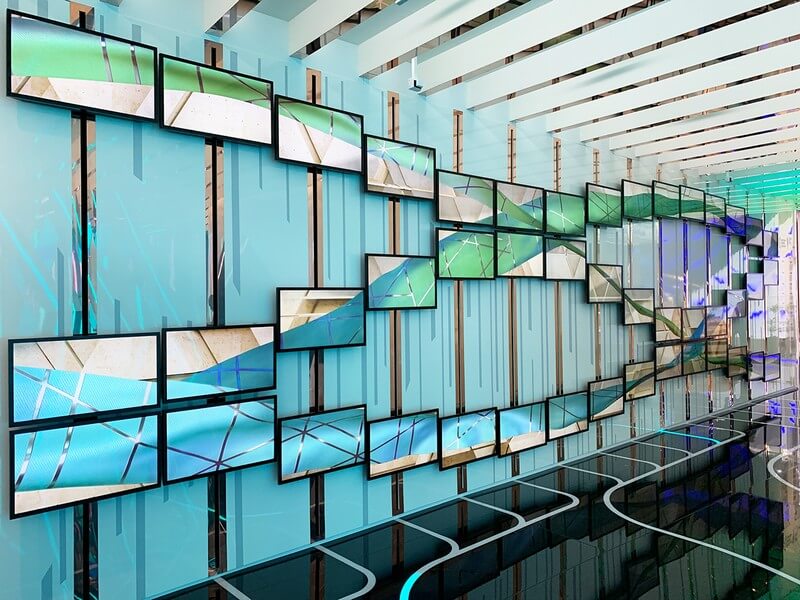This image depicts a captivating installation, likely located in an art gallery or showroom, featuring an array of high-definition TVs arranged in a meticulously designed pattern on a unique blue wall with vertical black stripes. These TVs, possibly numbering over 30, display smaller images that collectively create a larger, cohesive picture. The visual design features interconnecting green and blue sections resembling pipes or plant-like elements, which converge in the center of the installation, further accented by brown and purple hues.

The room itself is designed thoughtfully, with a glossy black floor adorned with white stripes that reflect the TV images above, enhancing the visual experience. The ceiling is distinguished by numerous white horizontal pillars, adding to the modern, open feel of the space. The overall effect is visually striking, combining technological and artistic elements to create an engaging and immersive environment.